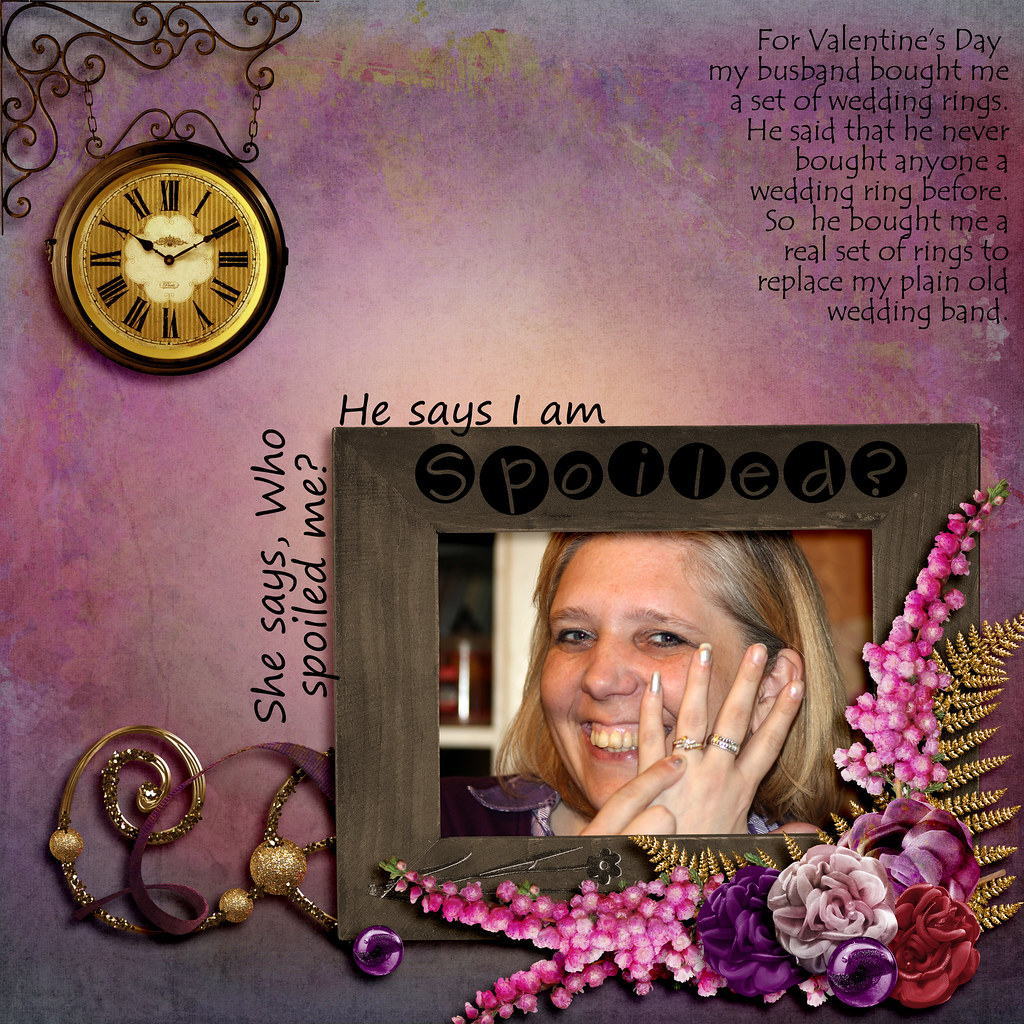The digital image features a primarily purple background with varying shades and a computerized design. On the top left corner, there's a gilded-looking gold clock. Dominating the top right section, text reads, "For Valentine's Day, my husband bought me a set of wedding rings. He said that he never bought anyone a wedding ring before, so he bought me a real set of rings to replace my plain old wedding band."

In the bottom right-hand side of the image, there’s a photograph of an older woman with dirty blonde hair, smiling and showcasing her new wedding rings. The photograph is inside a brown picture frame adorned with decorative elements. The frame's top side contains the word "Spoiled?" and surrounding text reads, "She says, who spoiled me? He says, I am." Positioned around the frame are various flower images in red, purple, and pink hues. The overall background color palette leans heavily on purples, enhancing the decorative, rich feel of the composition.